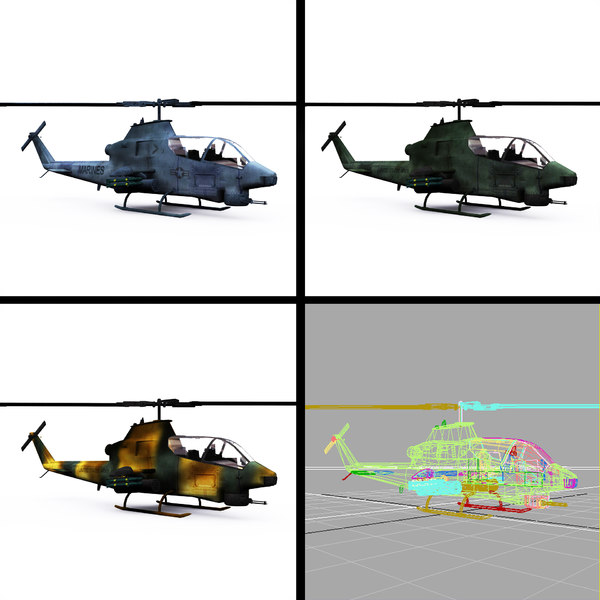This image is divided into four distinct sections, each featuring a helicopter. The upper left section showcases an older, worn grayish helicopter marked with a star on its side, seen from a right-side view displaying its window and cockpit. Adjacent to it, in the upper right corner, is a darker, military-style helicopter with a possible green and black camouflage pattern, presented from the same angle. The lower left section contains a yellow and black striped helicopter, viewed similarly from the right side. The lower right corner diverges from the photographic representations, displaying a schematic diagram of a helicopter against a solid gray background with a grid pattern. This diagram is color-coded in green, purple, blue, red, and orange, offering a detailed technical view. There is no text on the image, which is set against a white background, and the helicopters appear to be detailed, possibly military, unmanned models with front machine guns. The layout of the image resembles a window pane, suggesting a methodical comparison or an educational display.